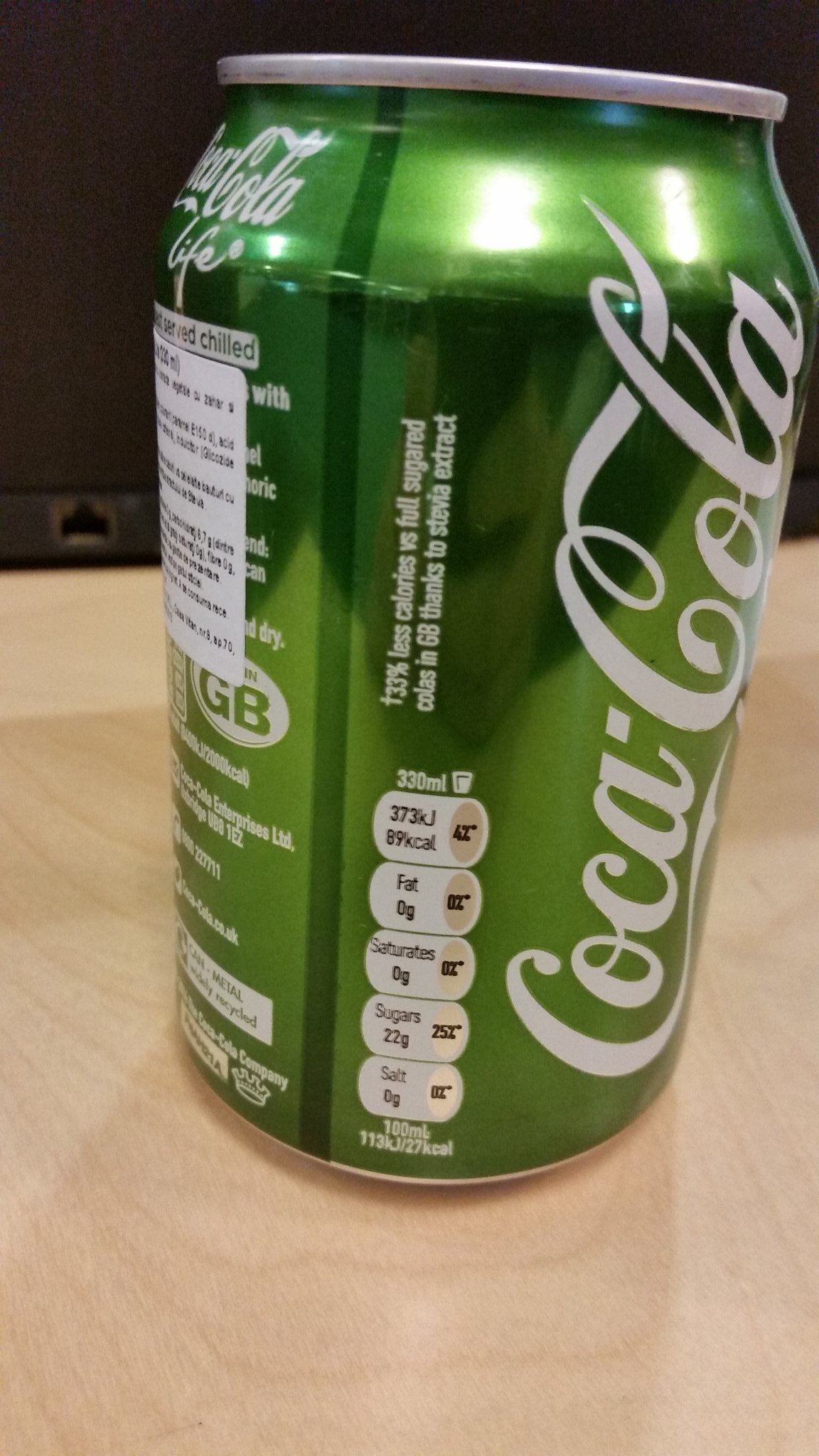This is a color photograph taken in a portrait orientation, captured indoors, predominantly featuring a green Coca-Cola Life can. The can deviates from the traditional red, white, and silver color scheme, presenting an intriguing variant. The side of the can faces the camera, showcasing some nutritional information in a compact infographic format. We can decipher key details such as 373 kilojoules, 22 grams of sugars, 0 grams of salt, 0 grams of saturated fat, and 0 grams of total fat in this 330-milliliter can.

The can has a silver top and bottom, and the Coca-Cola branding is written vertically in white text on the right-hand side, extending from the bottom to the top. Just above the main brand name, it reads "Coca-Cola Life" in white letters. Near the bottom center, additional text mentions “33% less,” although the text following this phrase is slightly out of focus. Further down, beneath the nutritional infographic, there are a series of square boxes filled with measurements and percentages—though some of these details are blurry.

A notable detail is the presence of a sticker partially wrapped around the left side of the can, likely an indicator of it being imported or a correction to a misprint. The sticker exhibits ingredients information but is slightly out of focus and not entirely readable in the photo.

The can sits on a tannish wooden table, with visible wood streaks and marks adding texture to the composition. The photograph also captures a reflection on the can's surface; the reflected image shows a person holding a phone, indicative of the photographer's presence. The can also reflects ambient light, adding to the visual interest of the image.